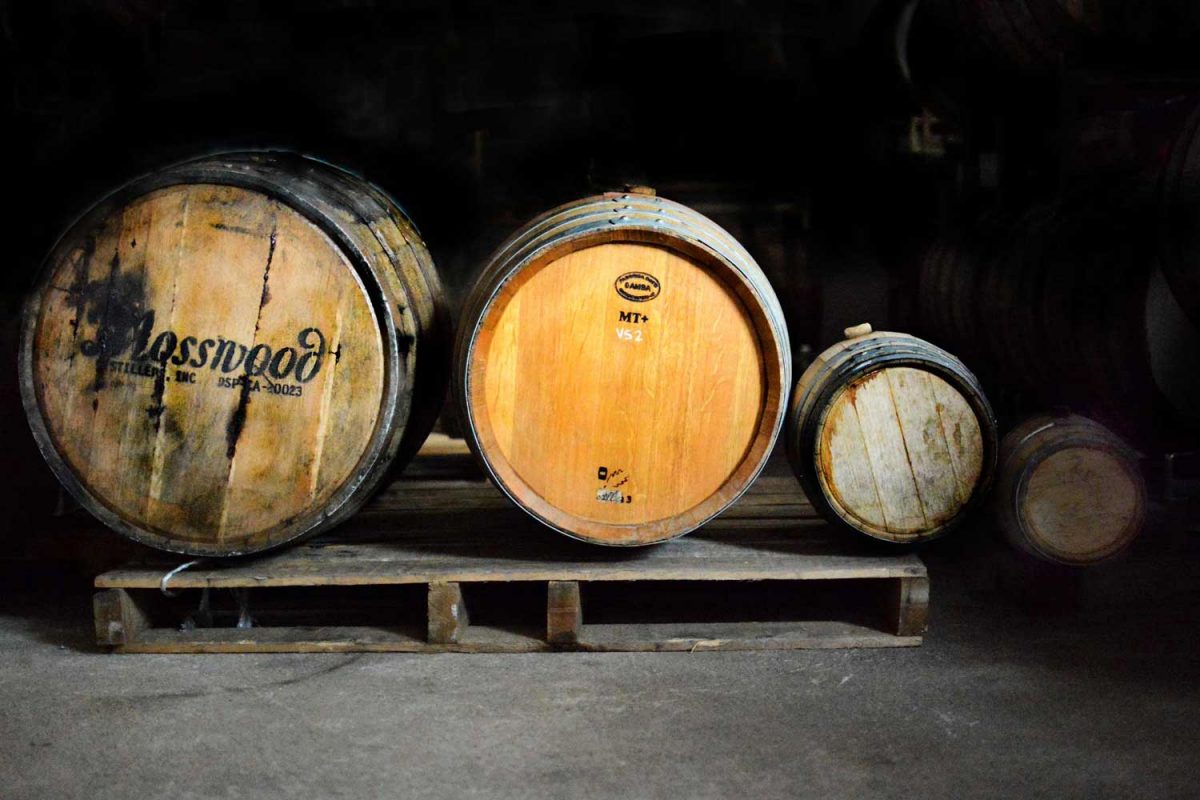The photograph captures a dimly lit cellar with a gray floor, featuring four wooden barrels arranged horizontally in a row from left to right, decreasing in size. The largest barrel on the far left, marked with the words "Mosswood Distillery," rests on a wooden crate and has a weathered, beat-up appearance, suggesting extensive use, possibly for aging liquor. Next to it is a slightly smaller barrel with newer, redder wood and reflective metal bands, indicating it is relatively fresh. The third barrel is smaller still, characterized by lighter, distressed wood. The smallest barrel, significantly tiny compared to the others, lies directly on the floor, not elevated by the crate. The setting is very dark, with the barrels gently illuminated by a soft light, highlighting the varying textures and conditions of the wood, and hinting at the aging process of the contents within them.